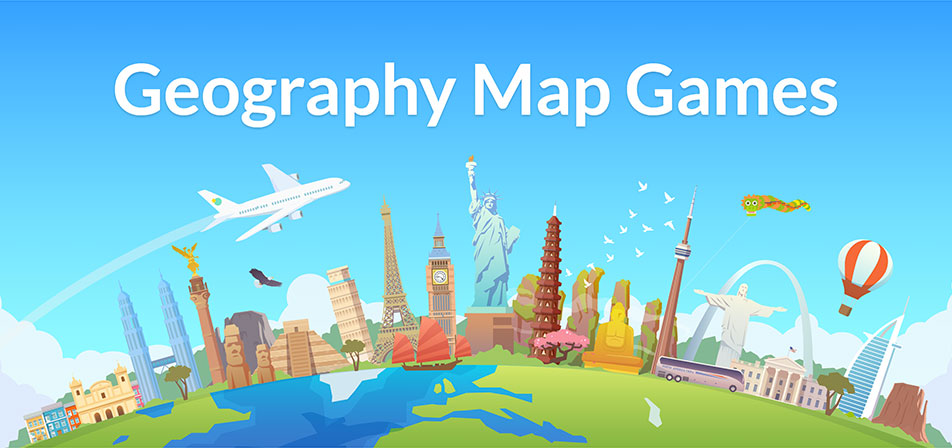This vibrant, digitally illustrated banner for "Geography Map Games" features a striking collection of world-renowned landmarks arranged in a whimsical composition. Set against a gradient sky that transitions from dark to light blue towards the horizon, the background includes wispy clouds and a large, white airplane leaving a vapor trail. The central focus is the Statue of Liberty, surrounded by other iconic structures such as the Eiffel Tower, Big Ben, the Leaning Tower of Pisa, Christ the Redeemer, the Burj Khalifa, and the Great Pyramid.

Below these landmarks, a partial globe suggests an interconnected world. Additional elements adding to the lively scene include a hot air balloon, a seahorse, a long tour bus, a boat in the ocean, and a whimsical dragon. The banner is topped with the title "Geography Map Games" in a white, sans-serif font with a soft blue shadow, emphasizing a lighthearted, educational theme.